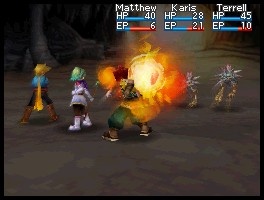This detailed caption combines the shared and key elements from each transcription:

"In this action-packed screenshot from a massive multiplayer online game, three players, identified as Matthew, Charis, and Tyrell, are engaged in battle. Each player’s status is displayed at the top right of the screen, with Matthew at 40 HP and 6 EP, Charis at 28 HP and 21 EP, and Tyrell at 45 HP and 10 EP. The characters, likely representing the players, are facing away from the viewer and combatting three obscured enemies. One of the enemies is casting a spell or attacking with fire, partially obstructing the view. The characters stand on brown stone within a forest-like environment, indicated by the trees in the background. The left character, possibly Matthew, is dressed in a blue outfit with blonde hair. The middle character, likely Charis, wears a white dress with green hair. The right character, presumably Tyrell, has green pants and red hair. Their names are clearly marked in white with black outlines for visibility against the dynamic backdrop of their intense confrontation."